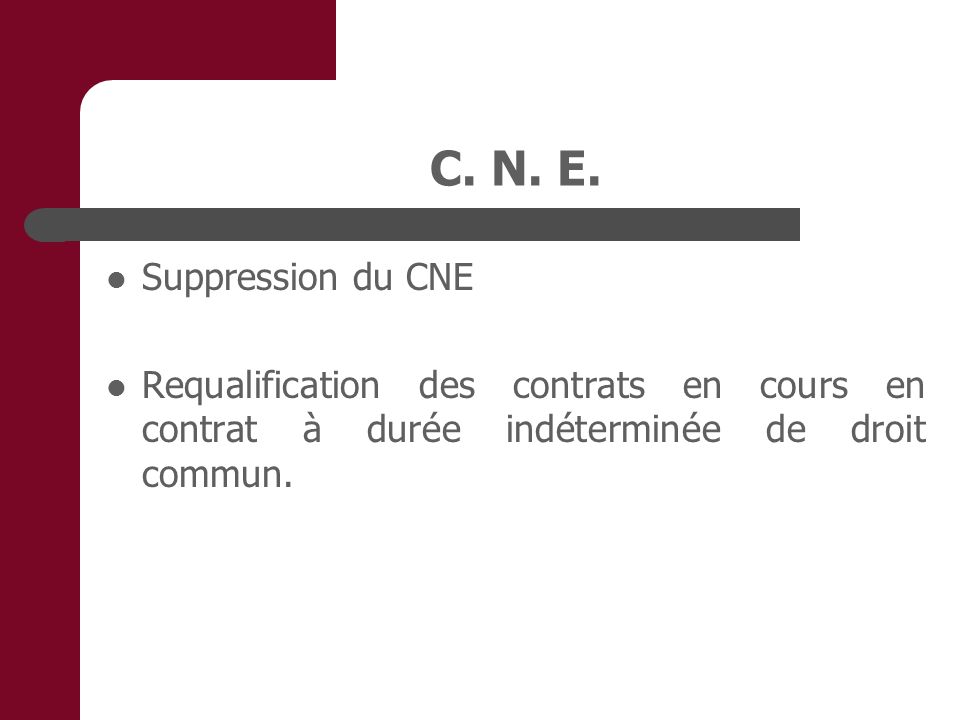The image features an informational text displayed in a foreign language, prominently centered against a nearly solid white background. On the left side, there is a rich maroon vertical frame extending from the top to the bottom and partially inward. The title "CNE" is prominently centered in gray text, underscored by a substantial gray line that stretches from the maroon section across the width of the image. Beneath this title, the content is organized into two bullet points marked by small gray dots. The first bullet point reads "Suppression Due CNE," and the second bullet point states "Requalification Des Contracts and Course and Contract A Duree Indetermine De Droit Commune." The text and elements maintain a balanced distribution, ensuring readability. The layout and design suggest that this could be part of a PowerPoint presentation slide. The color palette mainly comprises maroon, gray, and white.